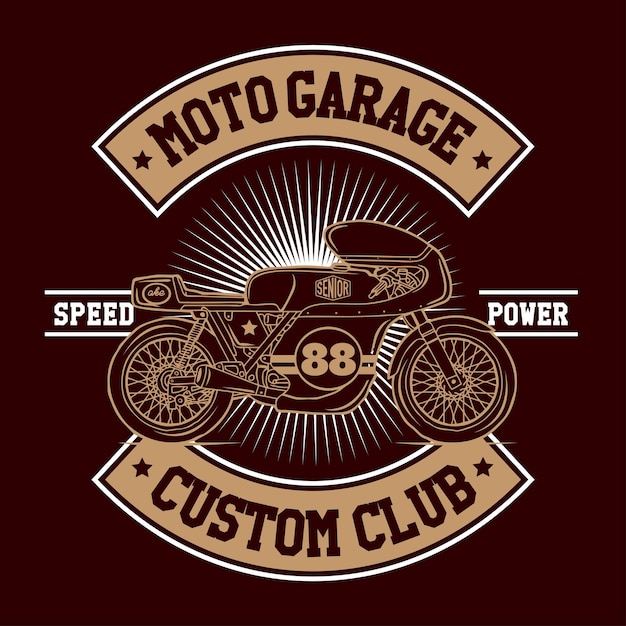The image features a detailed logo set against a completely brown background. At the top, there is a gold semi-circle with brown lettering that reads "Moto Garage," flanked by small stars on each side. Below this, a detailed digital illustration of a brown motorcycle, adorned with beige stripes and outlines, takes center stage. The motorcycle prominently displays the number "88" in gold on its side, along with the word "Senior." On either side of the motorcycle, white text labels "Speed" on the left and "Power" on the right. Beneath the motorcycle, another gold semi-circle frames the brown lettering "Custom Club." Additionally, a white, sunburst-like design encircles the entire logo, adding to its visual appeal.